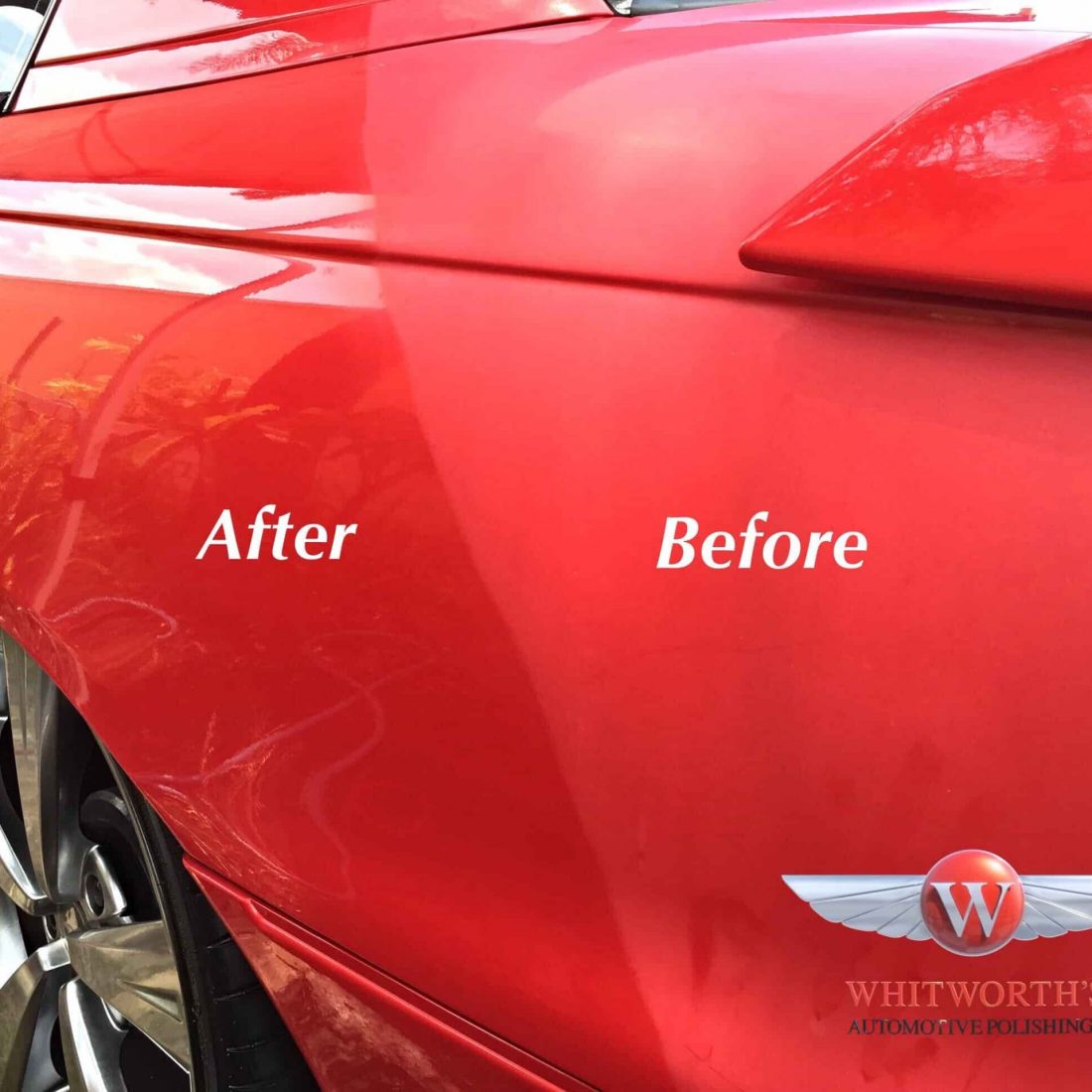This photograph showcases the back left quarter panel of a Candy Apple Red car, effectively illustrating a before-and-after polishing service from Whitworth Automotive Polishing Company. On the left side of the image, the quarter panel gleams brilliantly with shiny Candy Apple Red paint, and the word "After" is displayed in white lettering. Below this polished section, a black tire with a fancy aluminum hubcap resembling fan blades is visible. In contrast, the right side of the car is shown in a dull, matte finish, labeled "Before," and even shows a residual handprint in the paint. The bottom right corner of the image features a distinctive Whitworth emblem, consisting of a red orb with a white letter "W," flanked by white wings, and accompanied by the company name, "Whitworth Automotive Polishing," in pale red lettering underneath. This vivid portrayal highlights the transformative effect of the polishing service on the car's appearance.